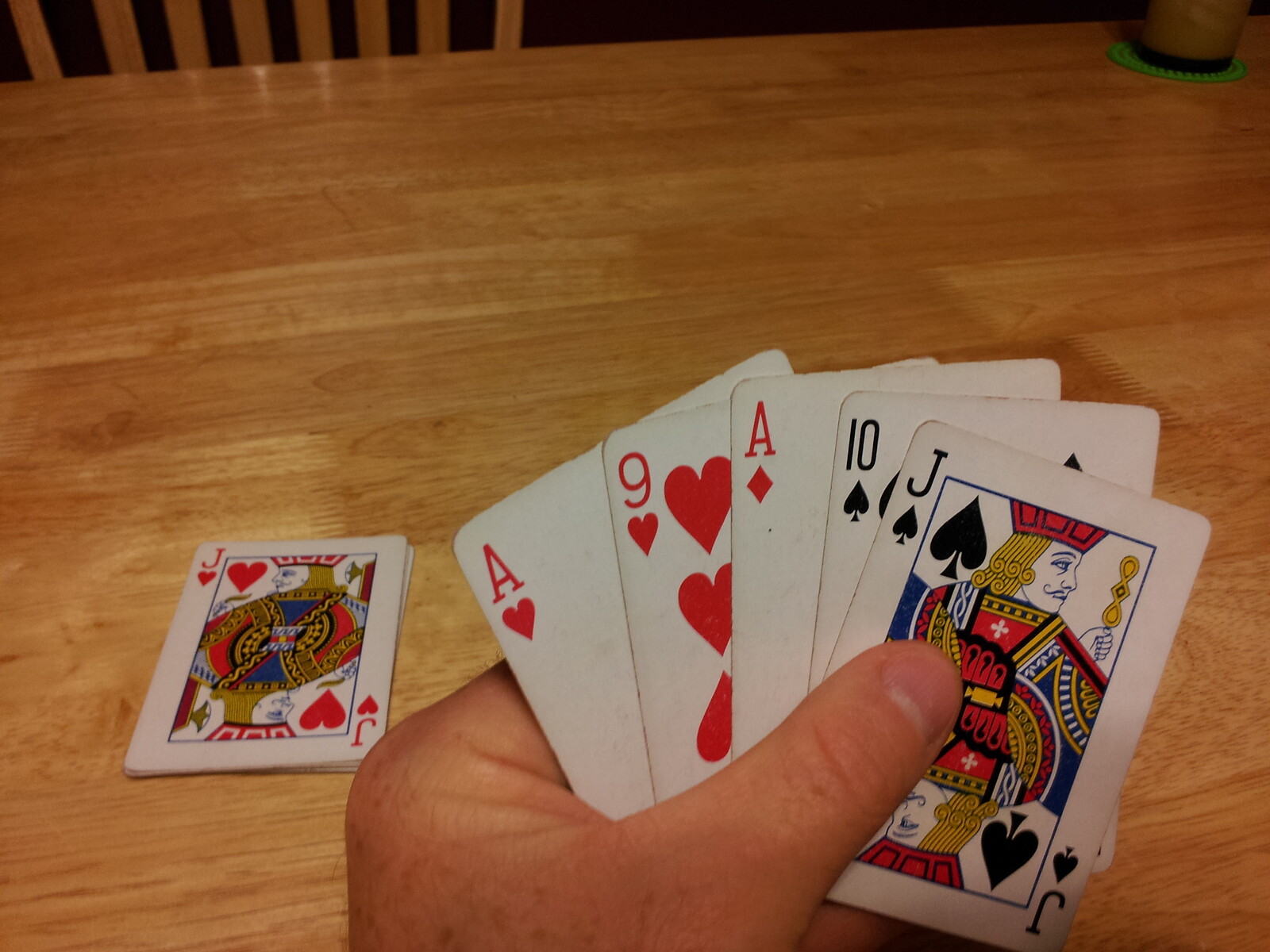This image captures an intimate scene of a card game in progress. Dominated by a large, light brown wooden table with visible grain patterns, the setting exudes a rustic charm. A partially visible wooden chair with its back showing is situated at the top edge, adding to the quaint atmosphere. Emerging from the bottom part of the frame is a hand holding a fan of playing cards, specifically the Ace of Hearts, Nine of Hearts, Ace of Diamonds, Ten of Spades, and the Jack of Spades. On the tabletop, slightly to the right, rests a small stack of cards, probably about five or six in total, with the top card being the Jack of Hearts, face-up. The absence of text directs all focus to the tactile, visual elements of the game, capturing a moment rich in anticipation or contemplation.